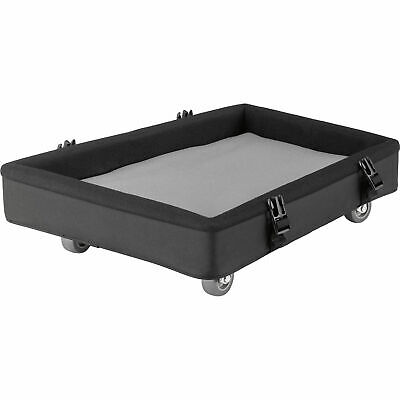The image depicts a black, rectangular rolling dolly designed for moving equipment. Its structure is short and flat with a lip around the edges, providing a shallow basin lined with a lighter gray material, set about two inches deep. The corners are rounded, and the dolly is edged with thick foam for added durability. It features four silver wheels made of hard rubber, allowing it to move in any direction. On both the left and right sides, there are black strap buckles for securing straps to hold items in place while in transit. The entire dolly is presented on a transparent background, emphasizing its use as a product image.